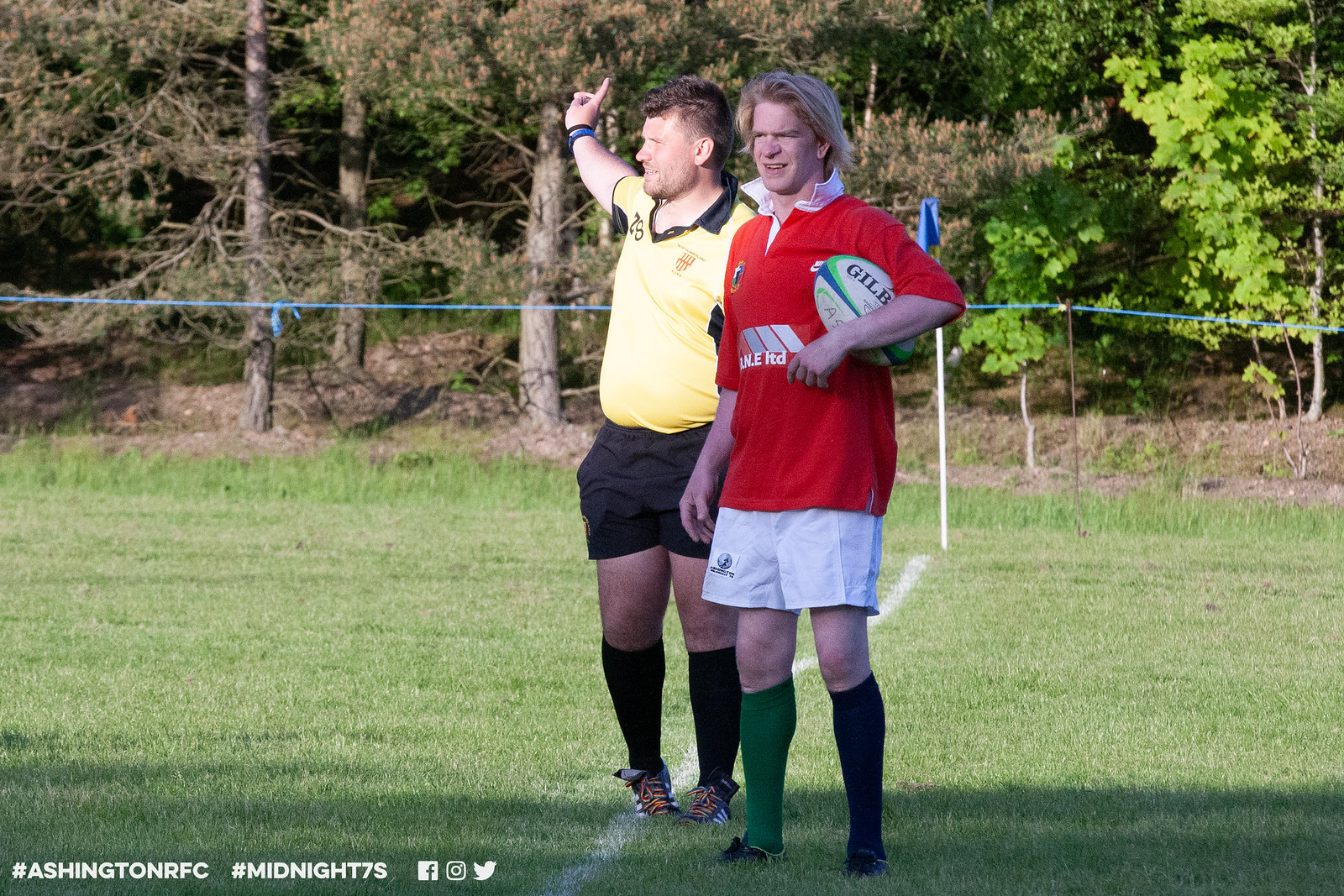The image captures two rugby players standing on a grassy rugby field, shown near a white boundary line that runs across the bottom of the frame. On the right is a player dressed in a red rugby shirt with a white collar, holding a white, blue, and green rugby ball under his left arm. He has blonde hair, white shorts, and different colored socks—green on his right leg and black-and-white on his left. His right arm hangs by his side, and he's gazing slightly to the right. To his left is another player wearing a yellow jersey paired with black shorts, high black socks, and a wristband on his right wrist. He has short brown hair and is looking to the left, with his right arm reaching behind him and his finger pointing upwards. The field is bordered by a fence with a bluish tape across the top, beyond which lies a dense forest of green trees. In the lower left corner of the image, hashtags #AshingtonRFC and #Midnight7S are visible, alongside Facebook, Instagram, and Twitter logos.